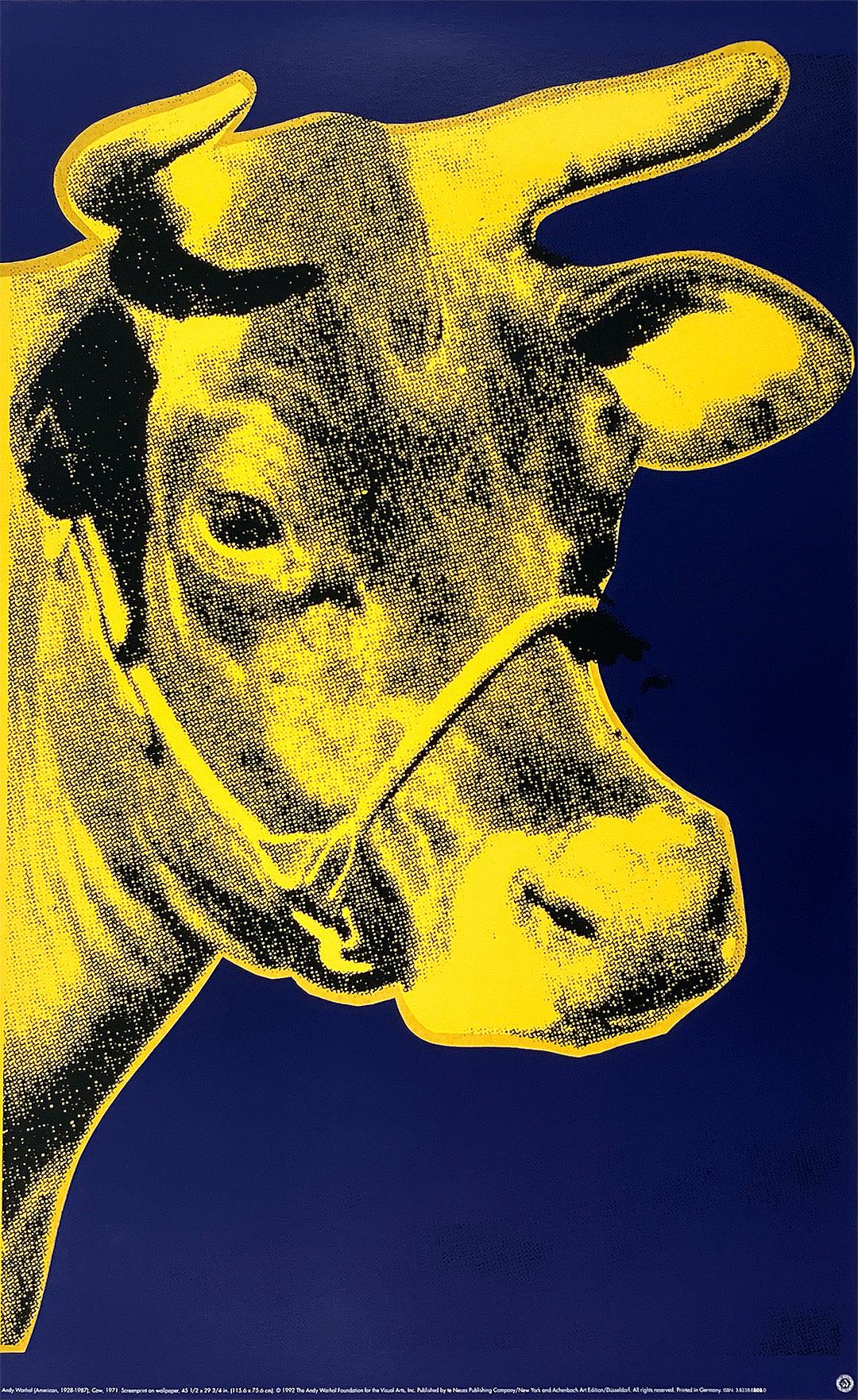The image is a vertically oriented, artist-rendered close-up of a yellow cow with gray and dark blue highlights. The cow's face and part of its neck are coming from the left side, with the background being a dark blue. Its two ears, two horns, and dark eyes are clearly visible, and it has a rope or harness around its nose that seems to be poking one eye. The horns curve slightly upward and toward the right. The cow's yellow coloring is prominent on its neck, the tip of its nose, inside one ear, and its horns. The rest of the cow includes brown and gray tones, with its appearance pixelated, giving it a CGI or dot-art feel. The cow is looking off to the right, and there is a small, unreadable white text along the bottom edge of the image, with a white symbol in the bottom right corner.